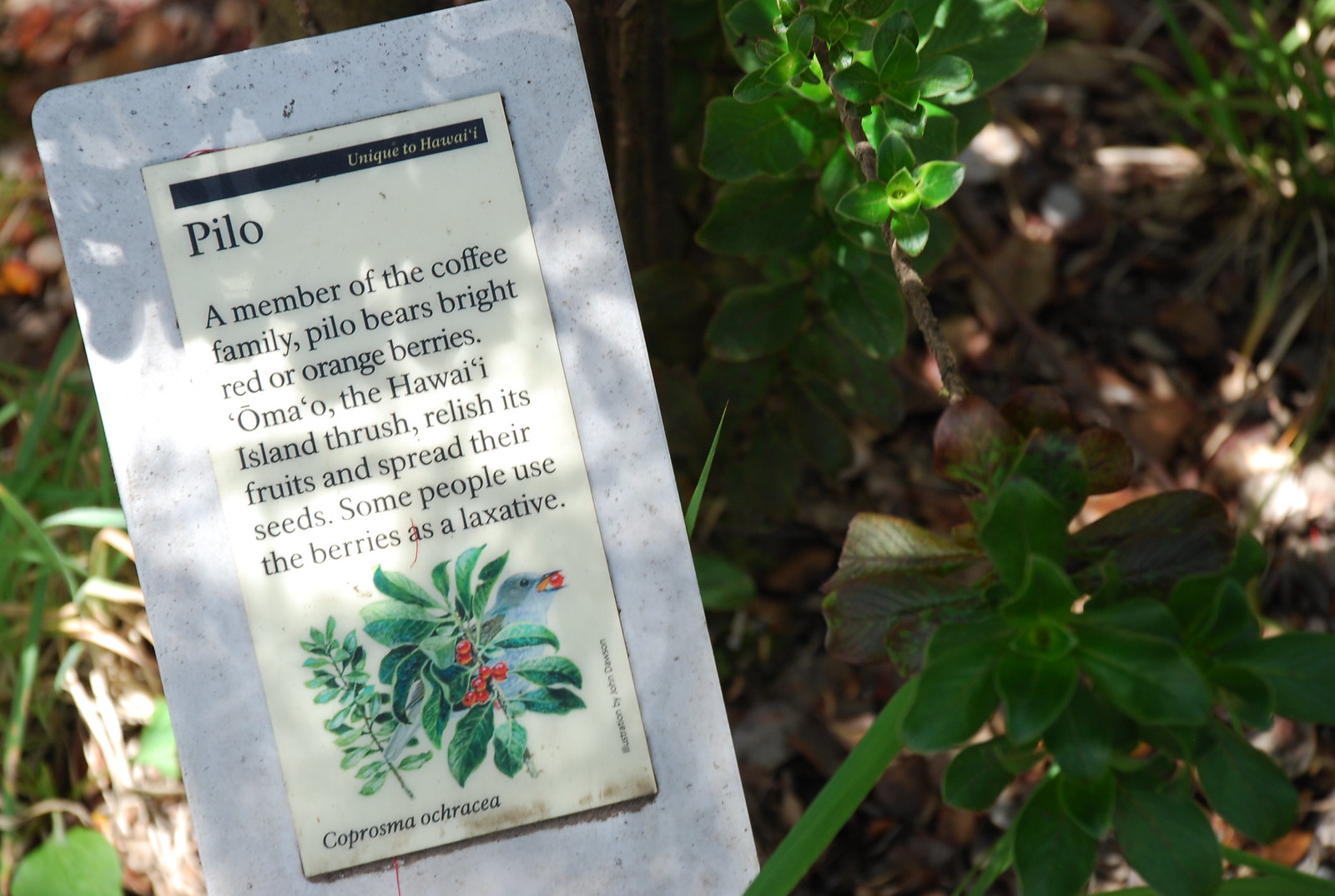The photograph, taken in full daylight, captures a garden area featuring several plant species. The main focus of the image is a particular plant called the pilo, which is notable for its association with the coffee family. A visible sign provides detailed information about the pilo plant, including its scientific name, Coprosma ochracea. The sign explains that pilo bears bright red or orange berries, though the actual plants in the photograph have not yet fruited. The berries are known to be relished by the Omao, the Hawaii Island thrush, which helps in seed dispersion. Interestingly, some people have historically used the berries as a laxative. Additionally, a full-color illustration on the sign depicts the pilo plant with its vibrant berries in bloom. Sunlight filters through the shadows, adding a natural and serene ambiance to the scene.